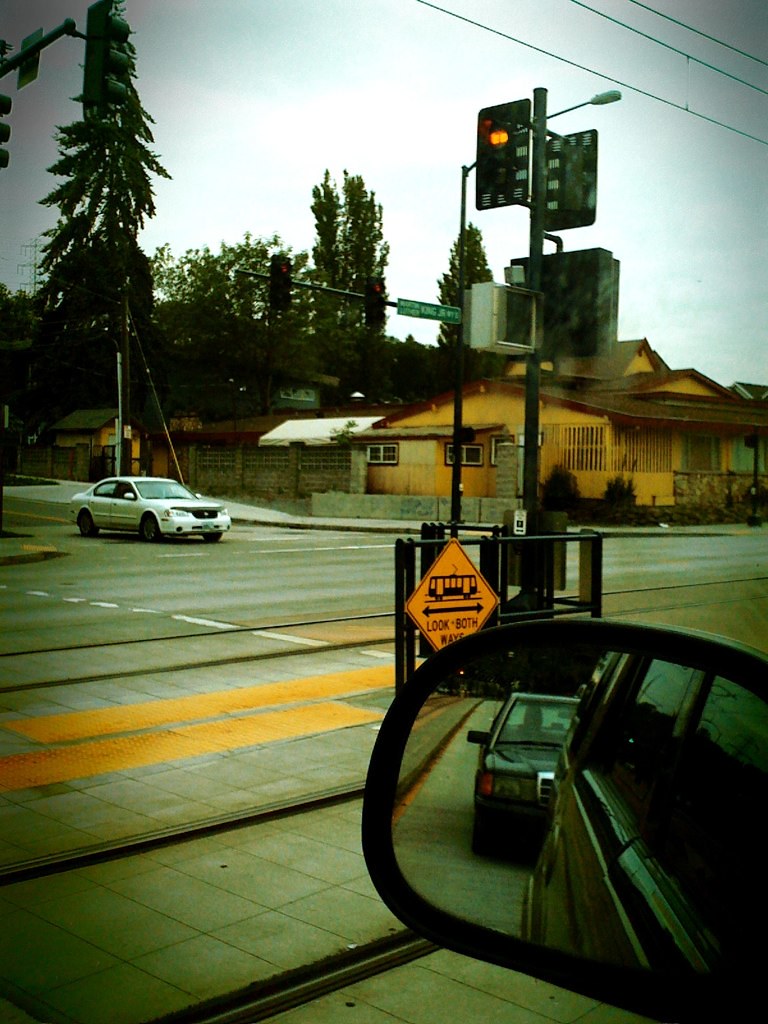This detailed photograph captures an intersection from inside a dark-colored vehicle. The bottom right corner prominently features the side mirror of the car, showing a dark-colored vehicle behind. Above the mirror, a sign with an orange triangle reads "Look Both Ways" and includes an illustration of a trolley car, indicating proximity to trolley tracks that run through the street. To the left, a white car is either stopped or preparing to enter the intersection. The intersection is marked by traffic lights, and the one facing the photographer is red.

The background reveals a light brown and yellow building with gray bricks and a reddish-brown roof, located caddy corner to the white car. The building features square windows and is set behind a brick fence. A street sign is visible, but its inscription is unreadable. The road, marked with yellow and white lines, is gray and smooth. On the left side of the frame, tall green trees stand against a light blue sky dotted with white clouds. The overall scene encapsulates a moment of stillness at a busy urban intersection, with the added complexity of trolley navigation.